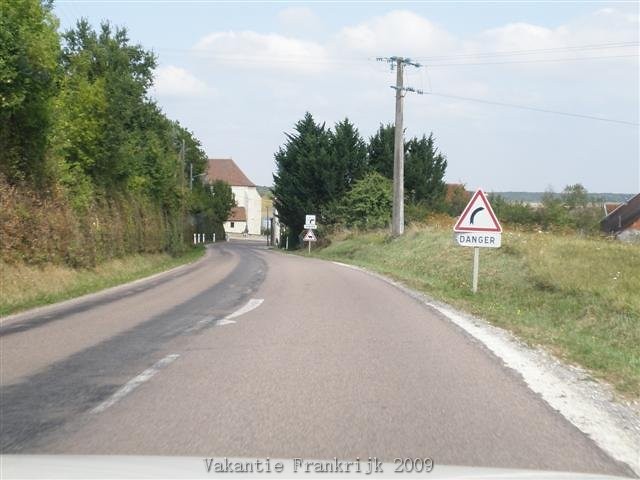The photograph captures a serene scene of a countryside road that curves to the right, typical of the English countryside. The road, possibly a two-track, is flanked by a blend of natural elements and man-made signs warning of the curve ahead. On the left side, a lush array of greenery including trees and overgrown weeds can be seen, with a black stripe of possible road repair stretching along its edge. Below this greenery, a curb is visible, demarcating the end of the road. To the right, the shoulder is covered with dying, yellowed grass and bordered by a well-manicured tree line. A telephone pole with wires crosses the image, emphasizing the rural setting.

The sky above is a striking blue, adorned with fluffy white clouds, adding a tranquil backdrop to the scene. Dominating the center, multiple road signs on white wooden posts with red triangles and curved shapes inside signal 'Danger' due to the upcoming bend. The signs increase in number as they recede into the distance, leading the viewer’s eye down the road.

At the end of the road, a cluster of white houses with brown rooftops and an old farm are nestled against the green landscape, marking the culmination of this picturesque journey through the countryside roads.